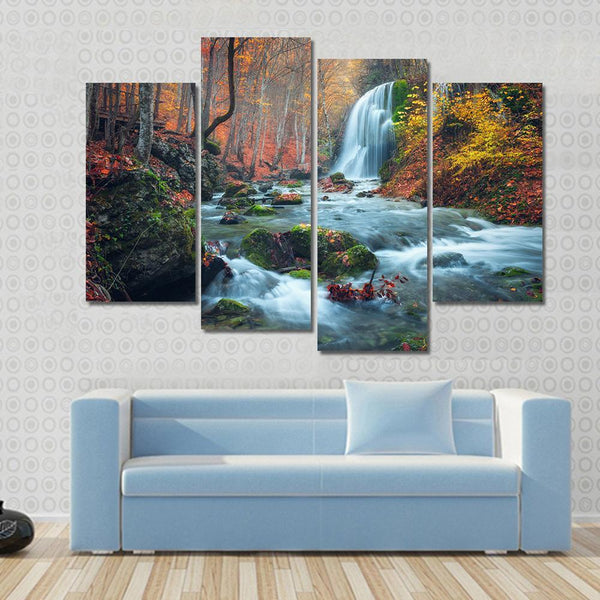The photograph captures an indoor living room setting with a light blue sofa, adorned with a single blue pillow, positioned on a light brown hardwood floor. The sofa sits directly against a wall covered in white wallpaper featuring gray circular patterns. On the left side of the sofa, there is a black electronic device, possibly a radio, stereo, or speaker. Above the sofa is a horizontally aligned quartet of framed images that together form a single, cohesive painting. The artwork depicts a beautiful autumnal outdoor scene with a river flowing through a forest, a waterfall, and rocks, with the surrounding trees showcasing vibrant orange foliage. An artificial light from above casts a white glow on the blue couch. The detailed composition and rich colors of the photograph evoke a tranquil and aesthetically pleasing environment.